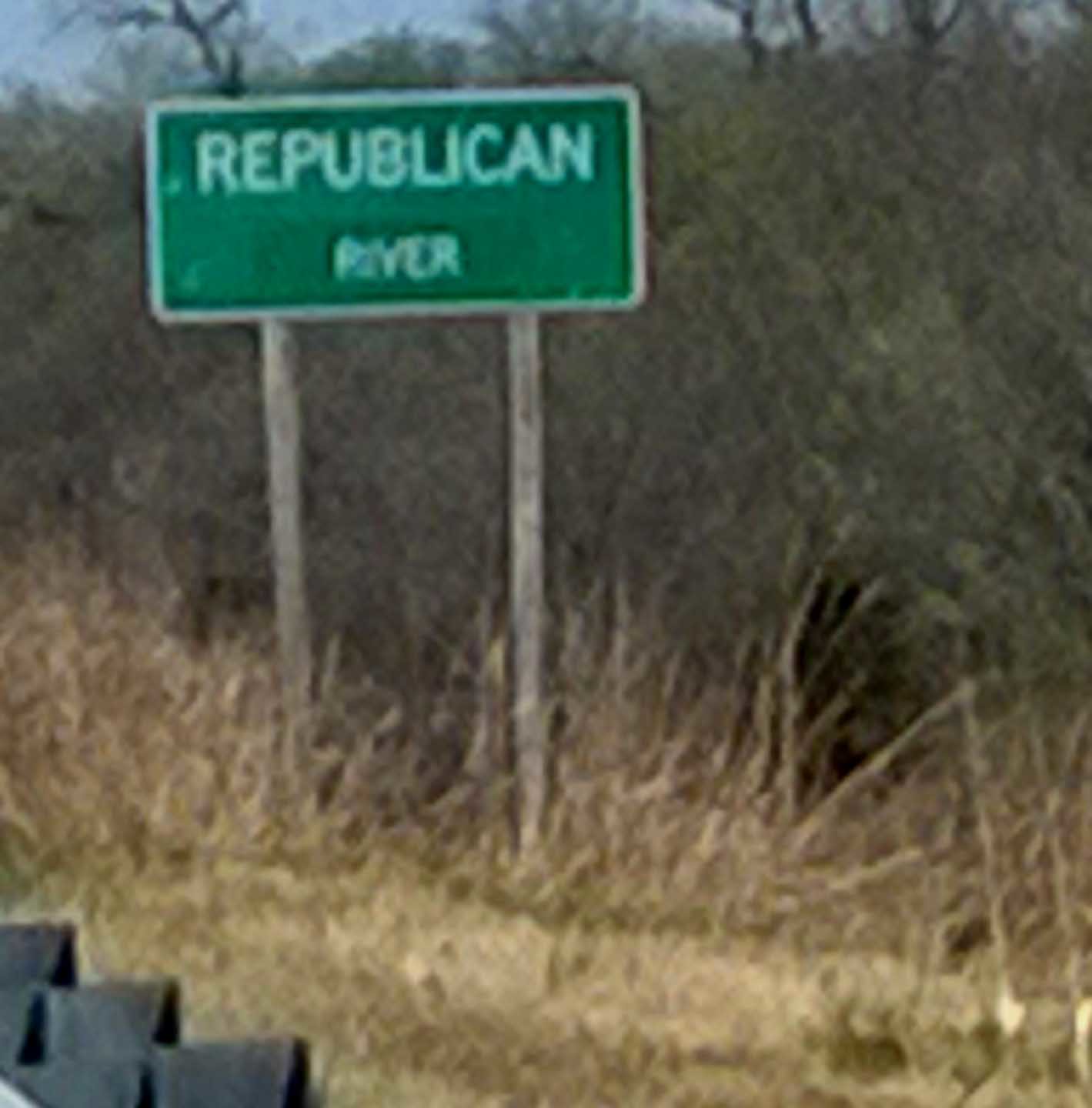This is an extremely blurred and low-quality photograph, likely taken at the side of a road in a natural setting. At the top edge of the image, there is a sliver of bluish-gray sky, though it's indistinguishable whether it is cloudy or not due to the blurriness. Below the sky, there is a row of trees with indistinct green, brown, and gray leaves, standing behind a slope covered with tall, dry yellow grass. In front of this tall grass is a shorter strip of green grass. Emerging from this grassy area is a green highway sign with white text that reads "Republican River." The background features dense shrubbery approximately 10 to 15 feet tall. There's also a dark object on the bottom left, possibly part of the highway barrier. The overall image quality is grainy, making it challenging to discern finer details, though it seems to have been taken on a relatively cloudy day.